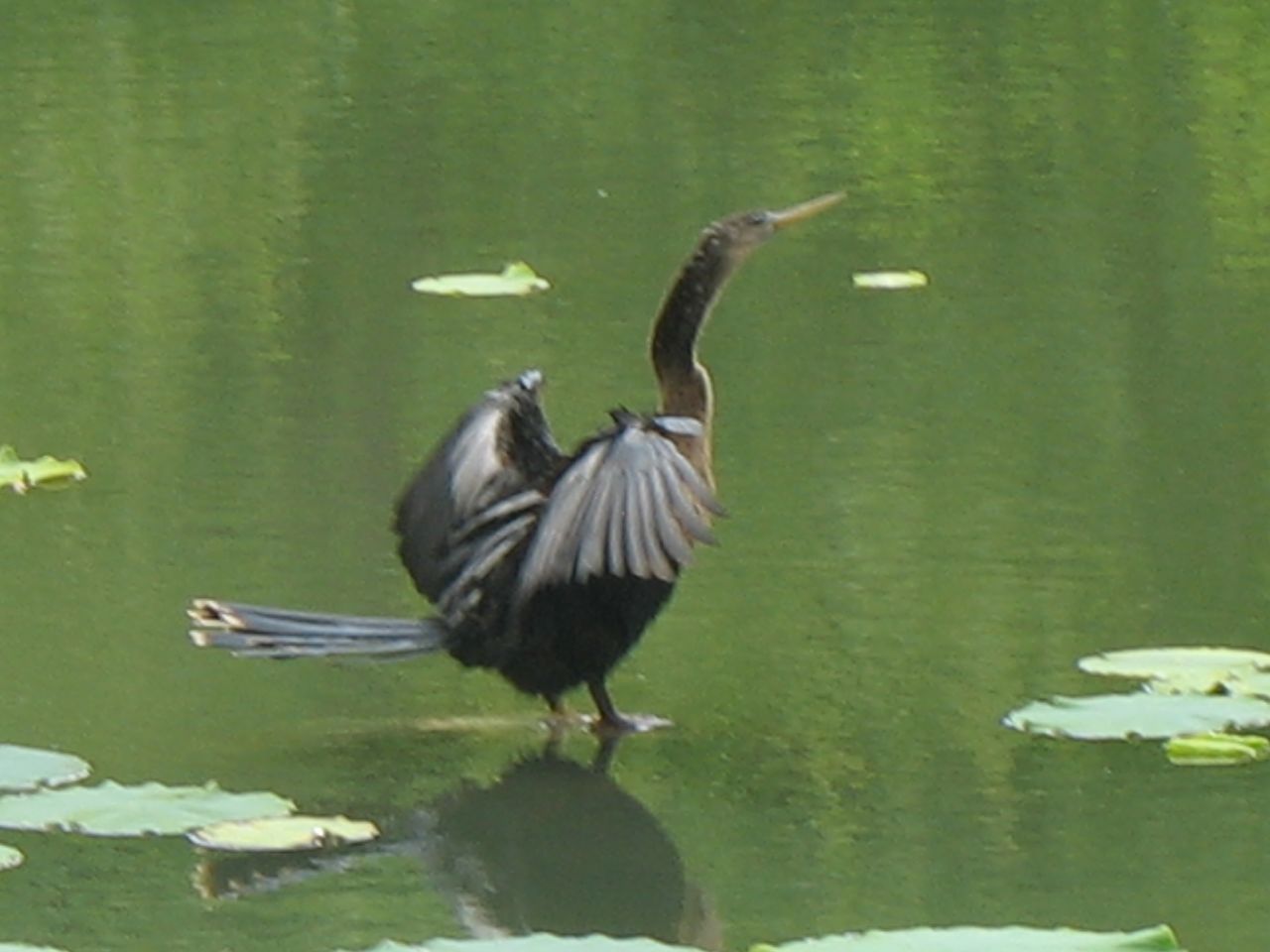The image features a duck of brown coloration with a long neck and a hint of white on its wings, standing in the center of a serene, green-tinted body of water. The duck is captured in a dynamic mid-wing span moment, either landing or preparing to take flight, with its tail lifted and neck extended, showing its right side profile. The tranquil water, possibly a lake or creek, is adorned with lily pads scattered around, particularly noticeable in the bottom left and right corners of the image. The setting is outdoors during the day, with no visible sky or sun.